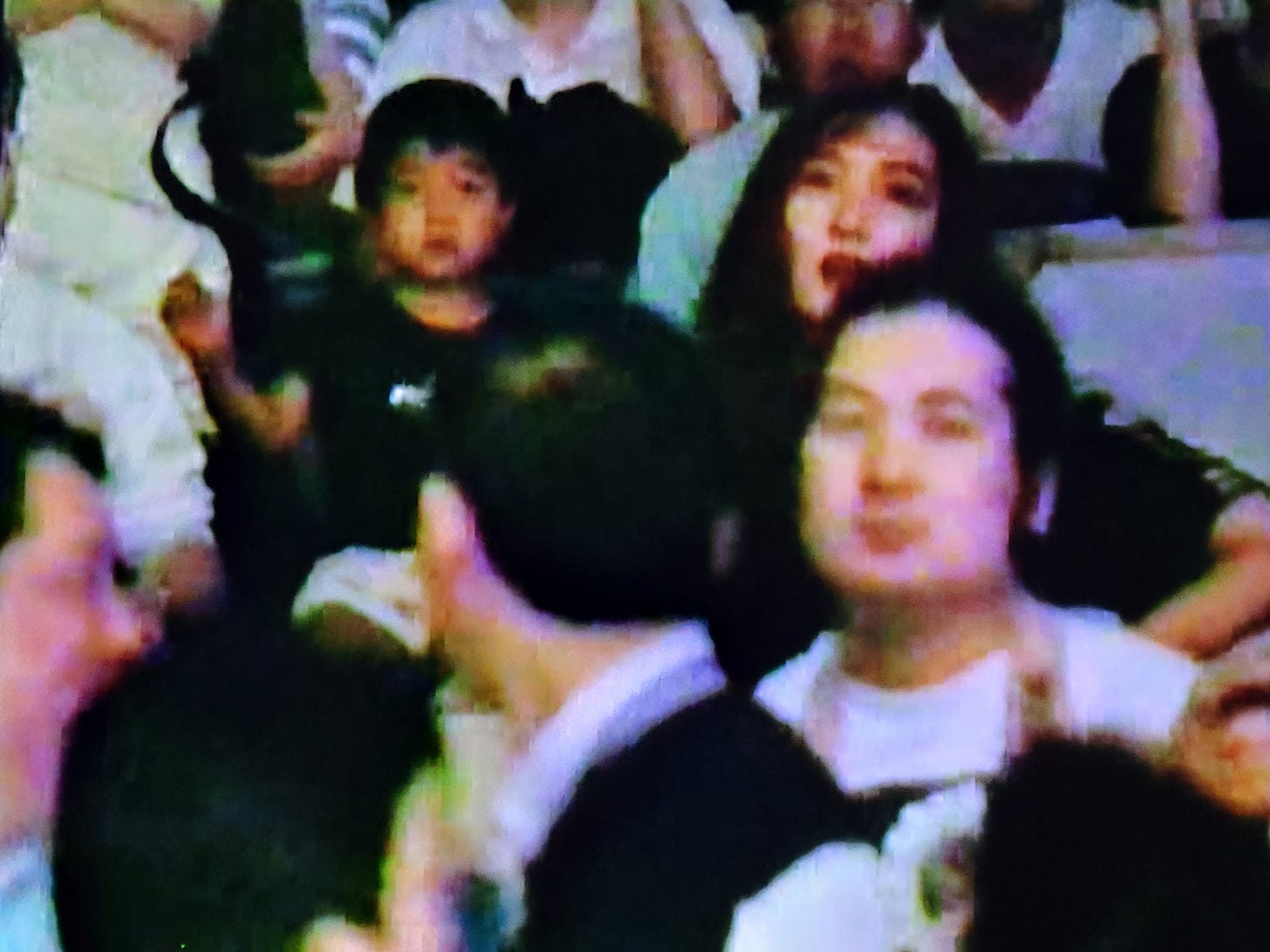A deliberately blurred and grainy photograph captures a dynamic scene, teeming with emotion and curiosity. At what appears to be a crowded event, a central figure of interest is an Asian toddler, about three or four years old, dressed in a black t-shirt and white shorts. The child stands with his right arm raised, his face reflecting a mixture of surprise and curiosity. Next to him, a dark-haired Asian woman, presumably his mother, is seated. Her open mouth and astonished expression, enhanced by her red lips, suggest she has just witnessed something startling. Another man, partially turned towards the toddler, seems to be smiling, though the blur makes his expression difficult to discern. Amid the assortment of people in various colorful shirts, one particular out-of-focus man in a white shirt stares directly at the camera, his features indistinct. The overall scene, though not sharply defined, is rich with a variety of emotions—from surprise to curiosity—capturing a compelling moment in time.